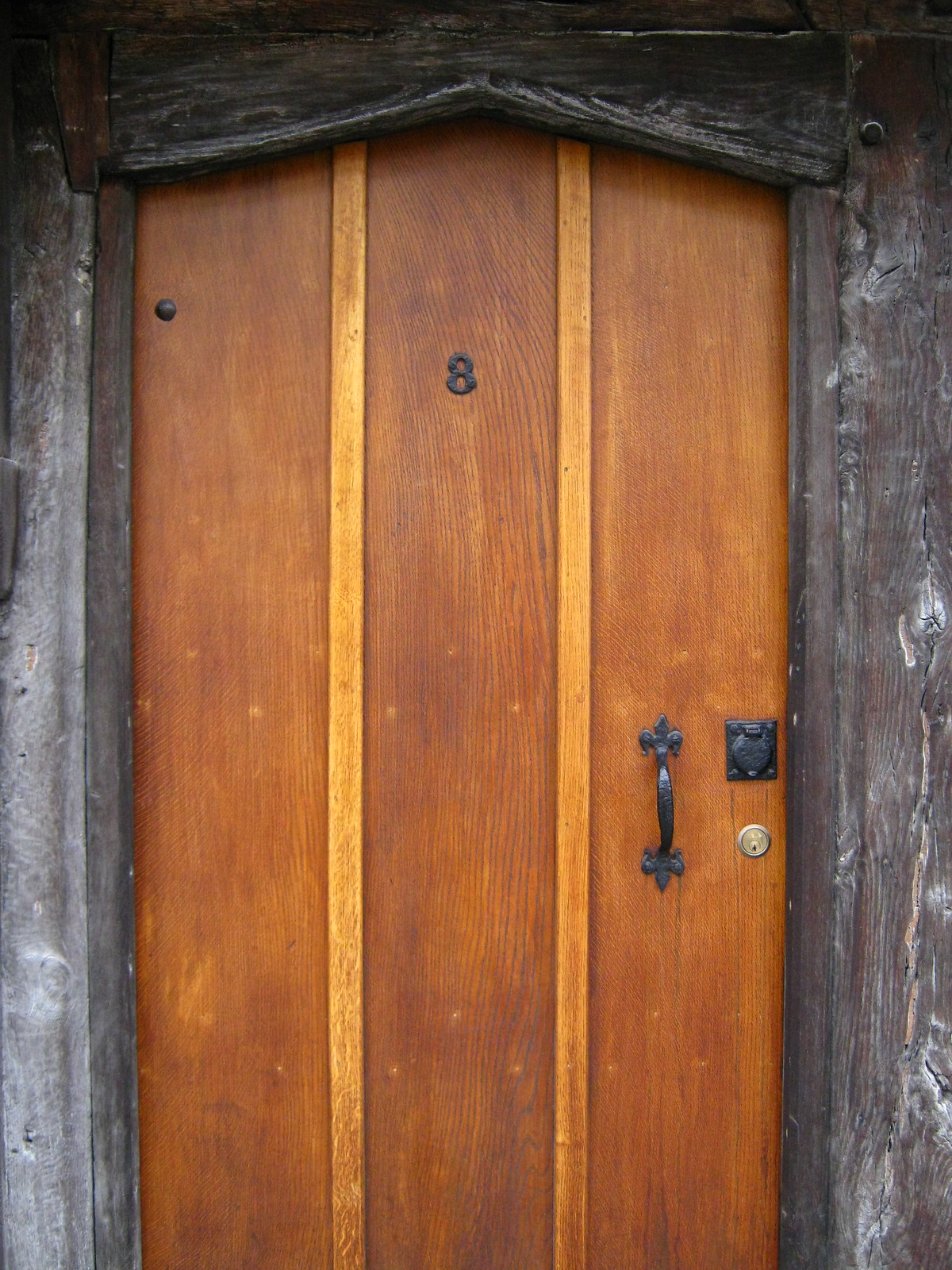This is a detailed close-up image of a large, mid-range stained wooden door, which exudes a sturdy and heavy-duty appearance. The door, displaying a visible wood grain, is flanked by two vertical wooden panels adding to its design appeal. Prominently positioned near the top center of the door is a small black number "8." Below this number, the door features a black wrought iron handle. Slightly above the handle is a small black square, a traditional lock, while beneath it is a more modern bronze keyhole. The doorway is encased in a darker, distressed wood frame that includes a subtle wooden arch at the top. The photo also reveals white spots on the lower left and right sides of the image, indicative of surrounding decor or structural details.